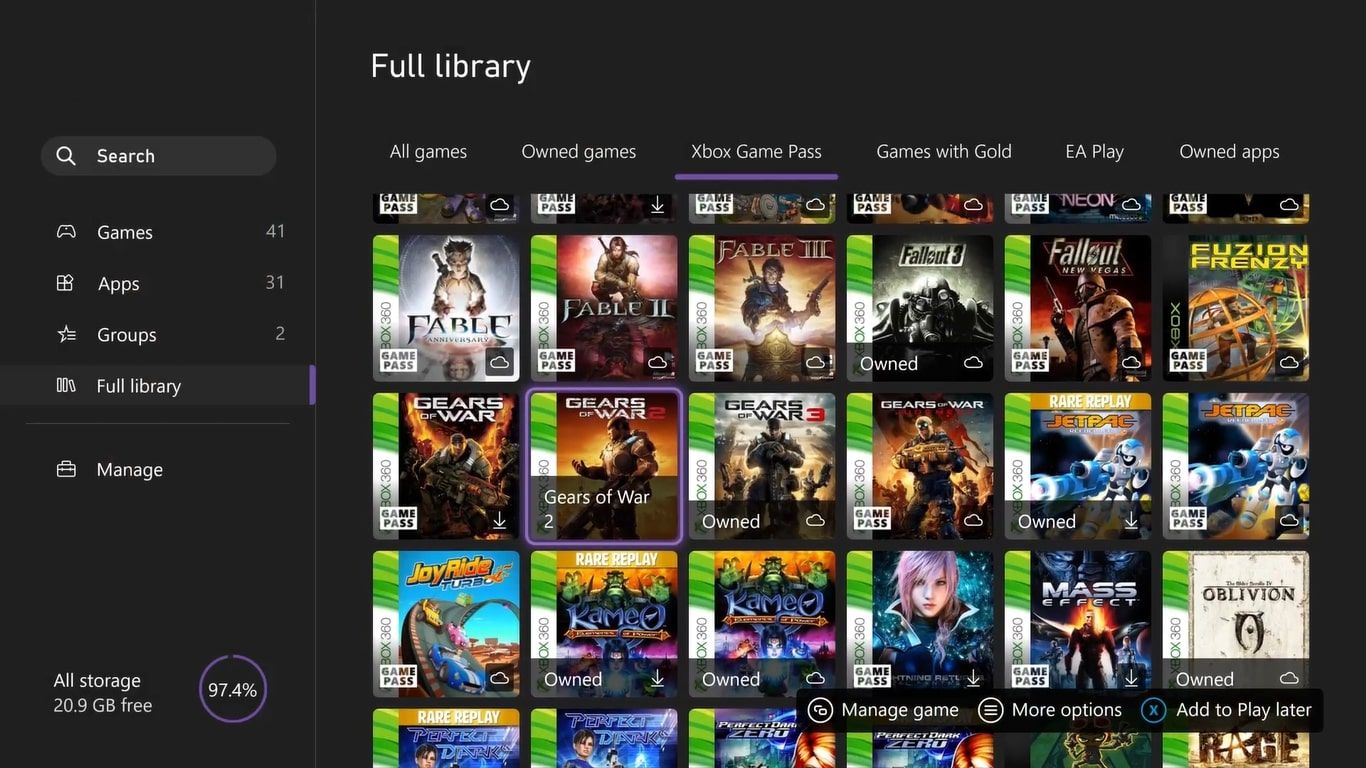The image displays a detailed interface of a gaming library. At the top, there's a header that reads "Full Library." Below this header, several categories are listed: "All Games," "Owned Games," "Xbox Game Pass," "Games with Gold," "EA Play," and "Owned Apps."

Further down, there is a grid showcasing various game titles, each represented by its cover art. The titles are arranged from left to right and top to bottom in the following order: 

- Fable
- Fable II
- Fable III
- Fallout 3
- Fallout: New Vegas
- Fusion Frenzy
- Gears of War
- Gears of War 2
- Gears of War 3
- Another Gears of War title
- Jetpack
- Another Jetpack title
- Rare Replay
- Joyride
- Camco
- Rare Replay (listed again)
- Regular Camco

Additionally, there's a game featuring a character with purple hair, identified as "Mass Effect," followed by "Oblivion."

On the left side of the interface, a vertical menu provides navigational options with the following entries: "Search," "Games," "Apps," "Groups," "Full Library," and "Manage."